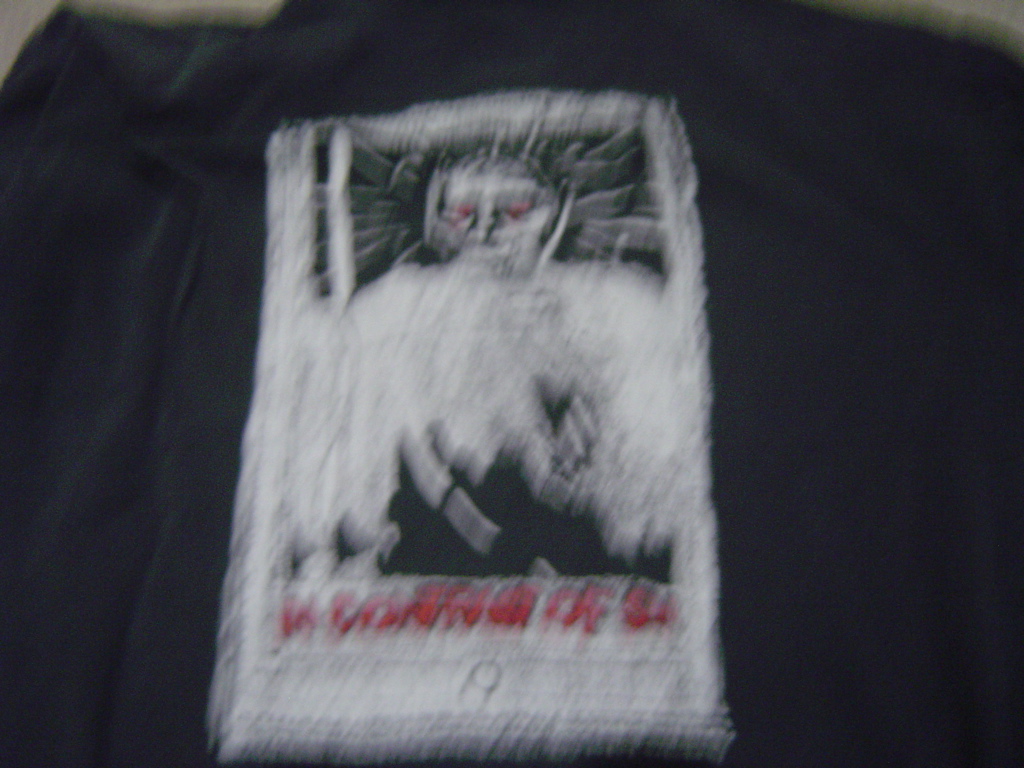This is a very blurry color photograph depicting what appears to be a black fabric garment, either jeans, a shirt, or a jacket. The fabric is slightly wrinkled, and at the center of the image, there is a large rectangular white patch. This patch features a demonic figure with red eyes, a prominent nose, and possibly wild black hair. The figure has black and white sharp images or designs protruding from behind its head, giving a slightly religious appearance. Dressed in white and black, the figure may also have some embroidered elements. Underneath the demon figure, there is some red script, which is illegible due to the blurriness. The entire graphic, including the white patch and red text, is somewhat crumpled, adding to the overall indistinctness of the blurry image.